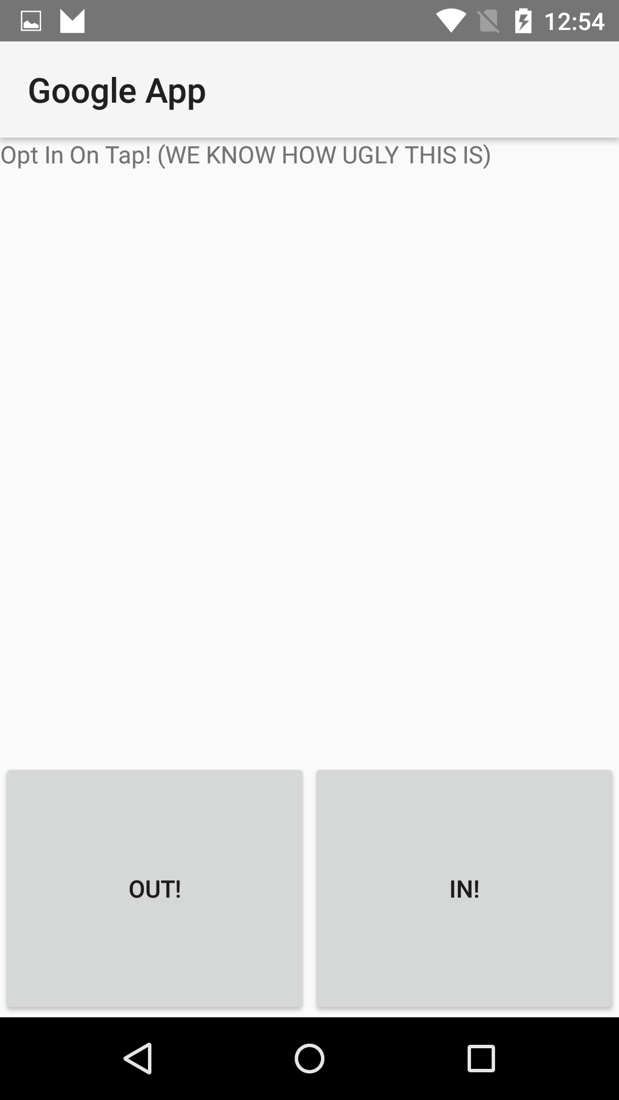The image displays a screenshot from a digital mobile device, primarily in off-white and gray tones. At the top of the screen, a gray horizontal bar is present, showcasing the battery life indicator on the far right and the current time. Directly underneath the gray bar, aligned to the left, black text reads "Google app." A horizontal gray line follows this text.

Below the gray line, in gray-colored text, the words "opt-in on tap" are visible, accompanied by an additional remark indicating dissatisfaction: "We know how ugly this is." This is followed by some empty space.

Towards the bottom part of the screen, there are two light gray square buttons. The left button displays the word "out!" with an exclamation mark, and the right button shows "in!" also with an exclamation mark. The very bottom of the screen features a black horizontal bar.